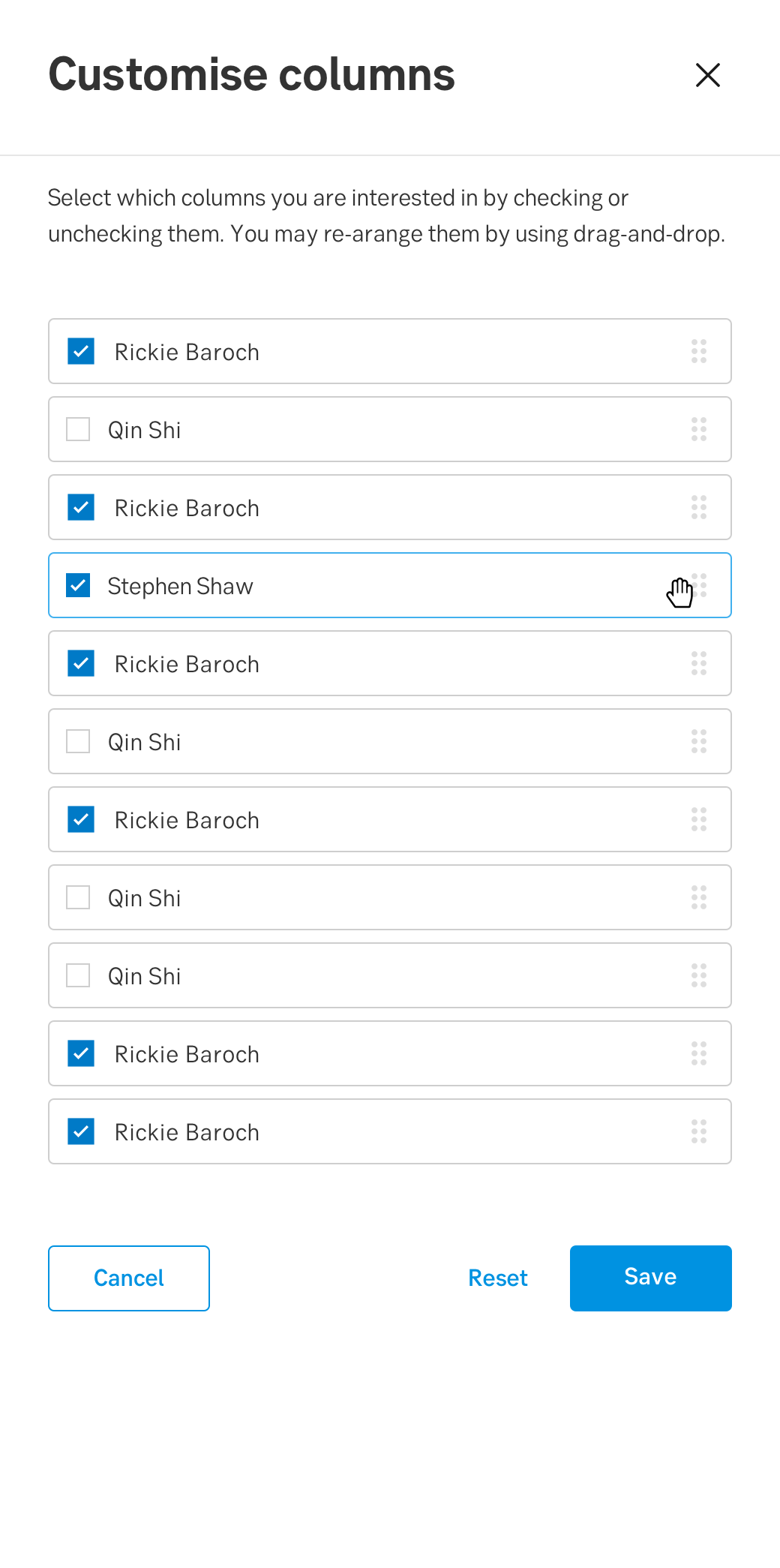A screenshot of a cell phone displaying a user interface for customizing columns. At the top, in bold, black letters, the title "Customize Columns" is prominently displayed, with an 'X' icon on the right to close the window. Below this header, a gray line separates the title from the instructions.

The instructions read: "Select which columns you're interested in by checking or unchecking them. You may rearrange them by using drag and drop." Beneath this instructional text, several rectangular blocks are arranged in a vertical list, primarily in gray and blue colors.

The list of columns includes:
1. A blue square with a white check mark next to "Ricky Baroch."
2. A gray rectangle labeled "when she."
3. A gray rectangle again named "Ricky Baroch," this time with a blue rectangle sporting a white check mark.
4. A blue square with a white check mark labeled "Stephen Shaw."
5. Another blue square with a white check mark again labeled "Ricky Baroch."
6. A gray square labeled "when she."
7. A blue square with a white check mark next to "Ricky Baroch."
8. Two consecutive gray rectangles labeled "when she."
9. Two blue squares, each with a white check mark, labeled "Ricky Baroch."

At the bottom of the interface, three action buttons are displayed. From left to right: a blue rectangle outlined in blue with the word "Cancel" in blue text, another blue word "Reset," and a fully filled blue rectangle with the word "Save" in white letters on the far right.